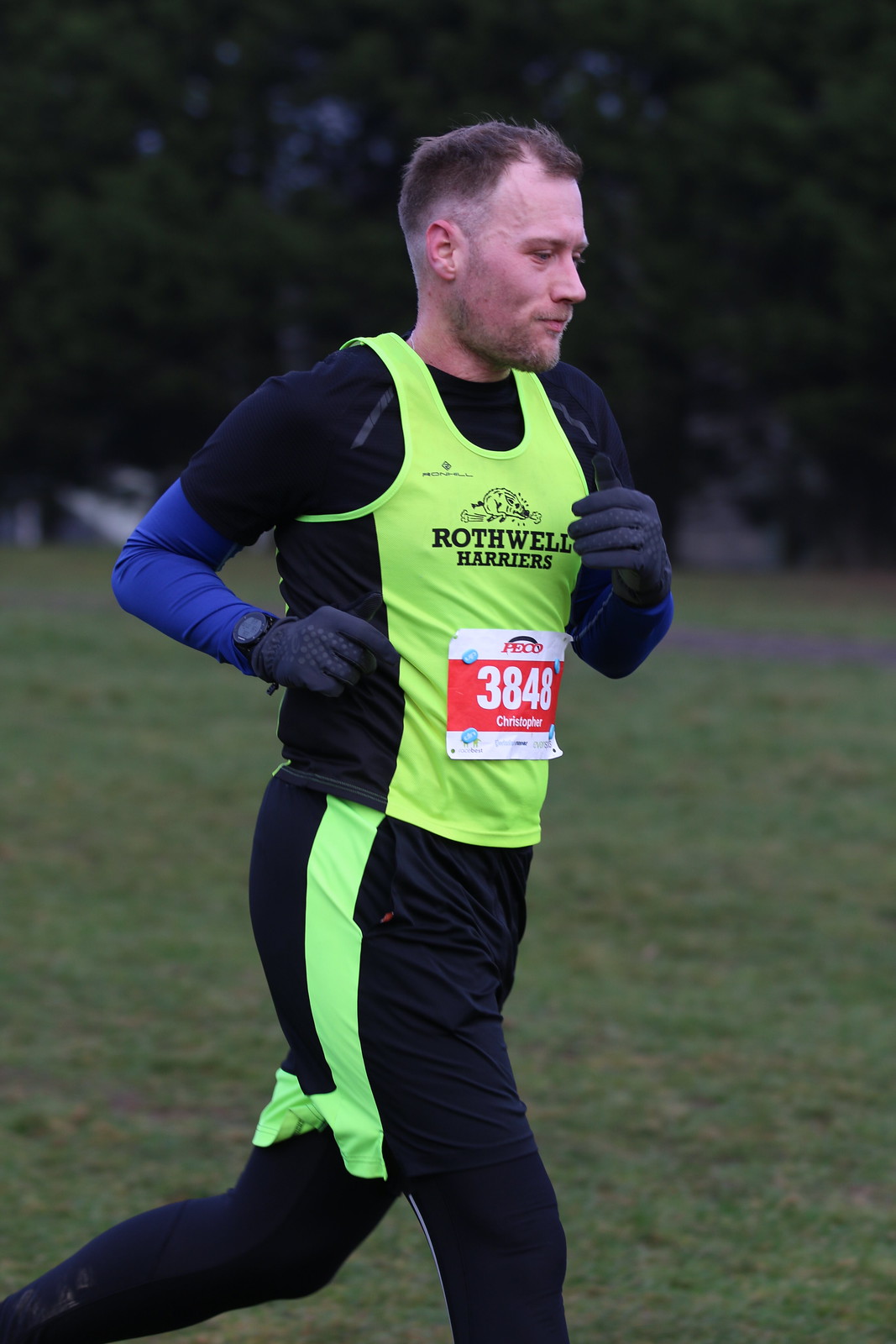The image captures a close-up of a man running in a race, likely cross-country, through a grassland with a background of tall, green trees. The runner has short brown hair and a five o'clock shadow along his jawline. He wears a layered outfit consisting of a long-sleeve Under Armour shirt and tights under a bright yellow tank top and black shorts with a yellow stripe on the right side. The tank top features the name "Rothwell Harriers" and a small logo resembling a mammal. His race number, 3848, is pinned to his chest. Additionally, the man is equipped with black gloves and a watch but no hat. He appears to be facing to the right side of the image as he runs.